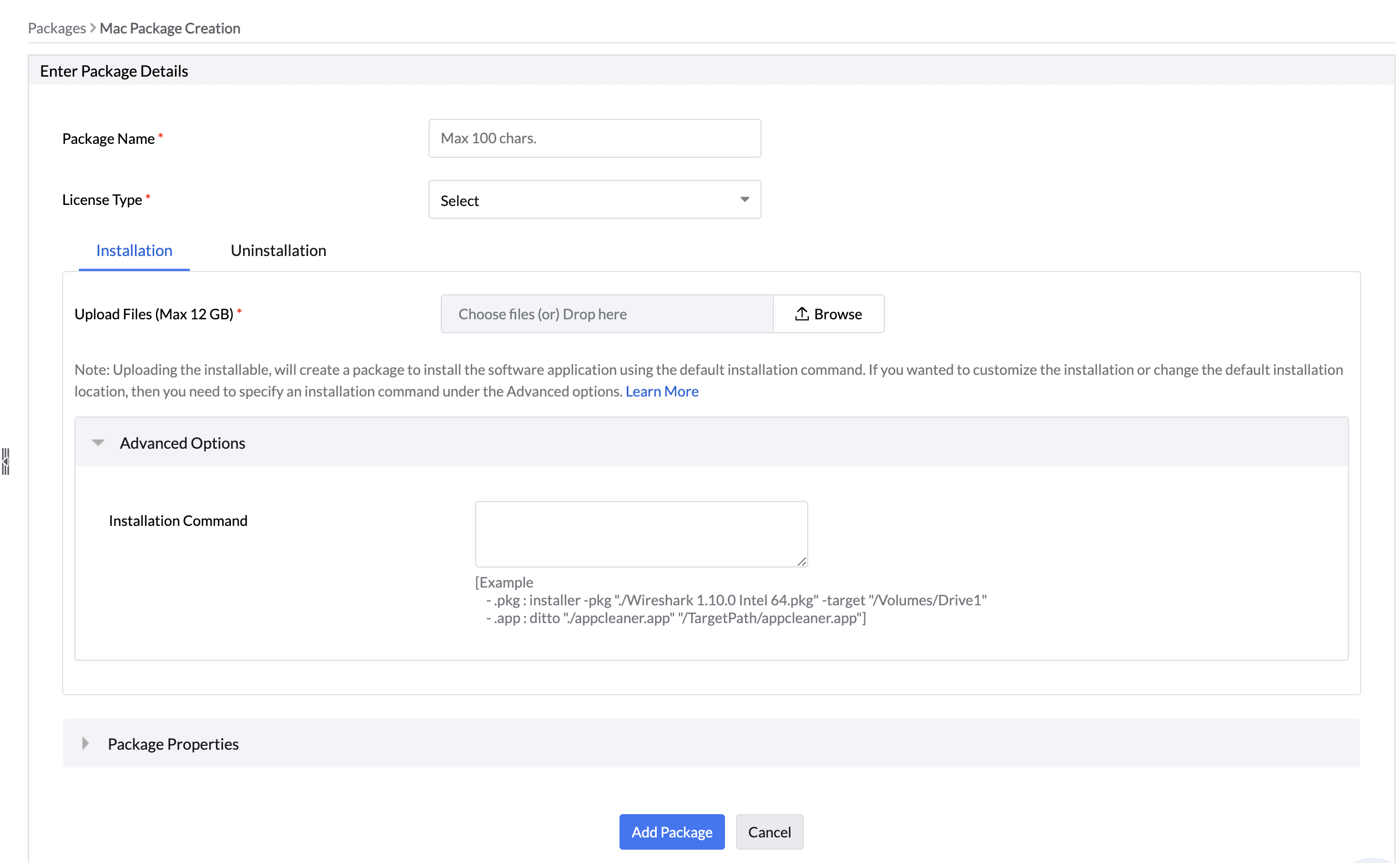### Detailed Description of the Image

The image depicts a user interface for creating a software package, presented in a structured and organized manner. 

**Header Section:**
- At the top of the interface, a clean white background features a grey text label that reads "Packages."
- Below this, in bold black text, there is the title "Mac Creation Package."

**Navigation Bar:**
- A thin grey bar spans horizontally, providing subtle separation from the header section.

**Content Section:**
- Against a light grey background, a black title reads "Enter Package Details."
- Below this, a labeled input field titled "Package Name" allows for entry of text, currently displaying "Macs 1000 Cares" in grey.

**Package Configuration:**
- The "License Type" section features a dropdown menu labeled "Select" in black, allowing users to choose the type of license for the package.
- Beneath this, a blue, underlined title labeled "Installation" is prominently displayed.
- Following this, in black text, "Uninstallation" and "Upload Files" are listed as subsections.
- "12 GB Macs" appears as the text beneath the "Upload Files" heading.

**File Upload Section:**
- A grey area for file uploads displays grey text that reads "Choose Files or Drop Here."
- A button labeled "Browse" in matching grey allows users to select files manually.
- An informational note in grey text provides guidance: "Uploading the installable will create a package to install the software applications using the default install command. If you want to customize the installation or change the default installation location, then you need to specify an install command under the Advanced Options."

**Advanced Options:**
- A blue text link labeled "or more" hints at additional configuration options.
- A gray box labeled "Advanced Options" in black provides access to these settings.
- A white background area marked "Install Command" allows users to input custom installation instructions.
- Within this section, there is an additional information box containing code, which is not described in detail.

**Footer Section:**
- At the bottom, a grey area labeled "Package Properties" in black provides space for additional package metadata.
- The image concludes with no further elements beyond this point.

This detailed layout encapsulates the various sections and functions available for users to interact with when creating a software package in the described interface.